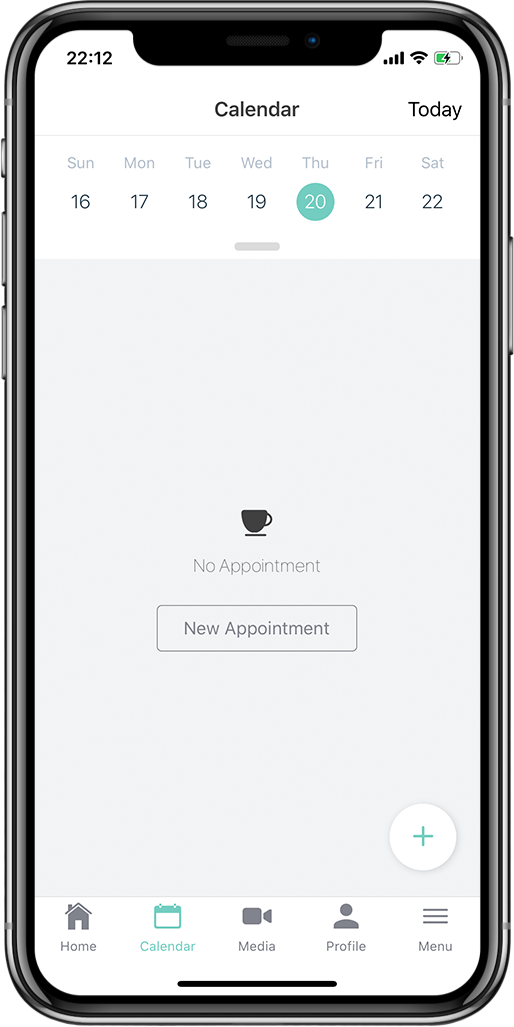A detailed screenshot showcasing an iPhone screen, highlighting its silver body frame and the blue top indicating the front-facing camera. The screen displays the calendar app. The status bar at the top reveals the time as 22:12, a fully connected Wi-Fi network, and a battery that is halfway charged. The calendar interface is open to the current date, which is circled in blue – the 20th of an unspecified month, falling on a Thursday. 

Within the calendar, the days of the week are listed alongside their corresponding dates: 16, 17, 18, 19, 20, 21, and 22. Below the current date, there is a notification area displaying "No appointments" with an icon of a coffee cup. There is a prominent plus symbol inside a circle at the bottom right, signaling the option to add a new appointment for Thursday, the 20th.

Additionally, the bottom of the screen features navigation options including Home, Calendar, Media, Profile, and Menu. The Calendar icon is highlighted in green, indicating the active view.